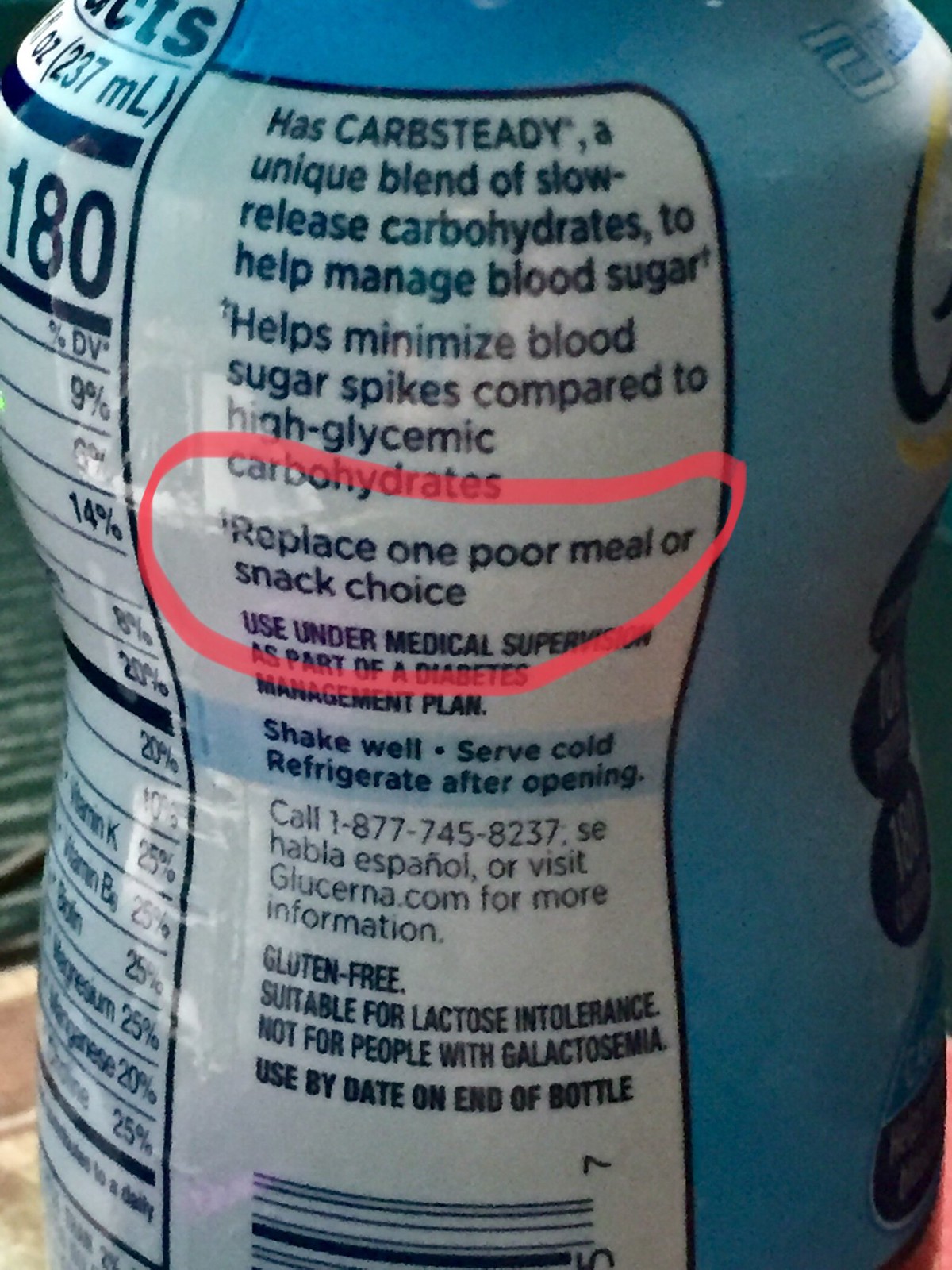The image depicts a blue bottle adorned with blueberry graphics visible along the right side. The bottle features a prominent label that is white with black trim, displaying detailed dietary information. At the center of the label, encased in a hot pink, fluorescent circle, the text reads, "Replace one poor meal or snack choice," suggesting the product serves as a meal replacement. Additionally, the label states the product includes "Carb Steady," a unique blend of slow-releasing carbohydrates to help manage blood sugar and minimize spikes, in comparison to high glycemic carbohydrates. Further down, it mentions that this product, originating from Lucerna, is gluten-free and suitable for individuals with lactose intolerance, though not intended for those with glass wall conditions. Users are advised to use this under medical supervision as part of a diabetes management plan.